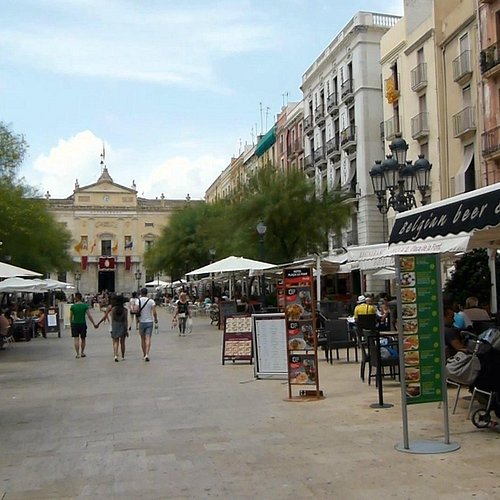The vibrant daytime image captures a bustling city market street, framed by large multi-story buildings on either side. The paved road, lined with various stalls to the right, leads the eye to vivid splashes of colors—yellows, greens, reds, blacks, whites, beige, and tans. These stalls, accompanied by signage indicating their wares, create a lively atmosphere with street lamps and restaurant menus adding to the urban charm.

A mix of locals and tourists, some with backpacks or purses, wander the streets. Among them, a couple holding hands adds a touch of intimacy to the scene, while others are seated at outdoor seating areas. The left side of the image prominently features some seating areas in front of another building at the center.

Lush green trees interspersed throughout the street add vibrancy against the palette of beige and white buildings. High above, a blue sky with white clouds stretches out, and a notable black flag with "Belgian beer" flutters near one of the stalls, hinting at the variety of offerings available in this area. The street surface, likely composed of gray stone, completes the picture of this dynamic urban market, beckoning visitors to explore and enjoy the myriad experiences it offers.